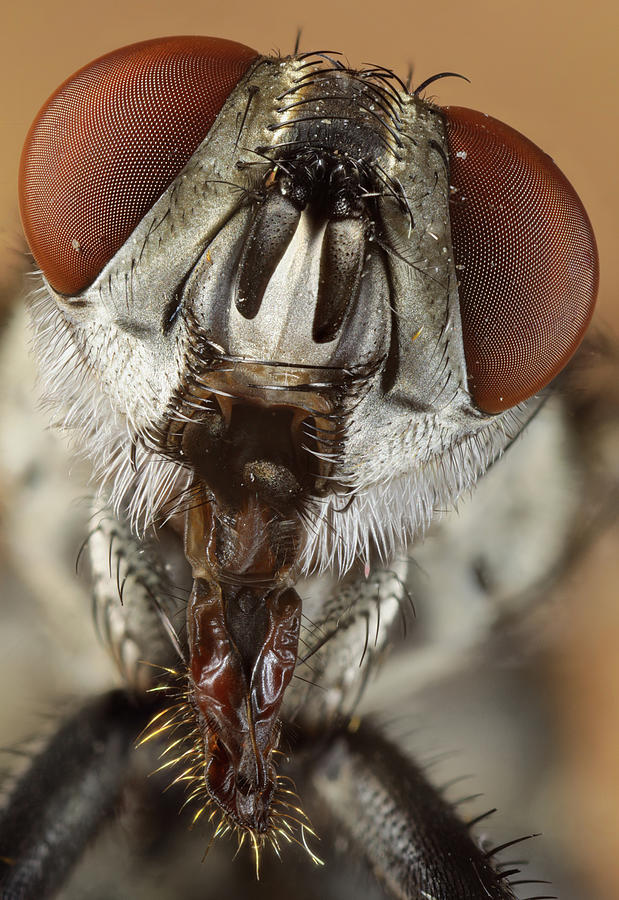This image is an extremely detailed, close-up photograph of a housefly's face. The photo appears to be so intricately detailed that it seems almost computer-generated. The face is shaped like an upside-down triangle, and the head is primarily focused in the frame, with the blurry, brown-tinged body visible in the background. The fly's eyes are notably large and red, featuring a mesh-like pattern made up of several tiny holes with some dirt or debris scattered on them. Covering the head are hair-like strands, adding to the realism. The mouth area is brown and includes long pincers with spiky projections, resembling small teeth. There are additional spiky elements scattered around the insect's face. Beyond the mouth, sharp parts of the body, possibly legs, can be seen, which are covered in black and gray hairs. The overall impression is that of a very close and vivid depiction of the fly's head, amplifying its alien-like and intricate features.